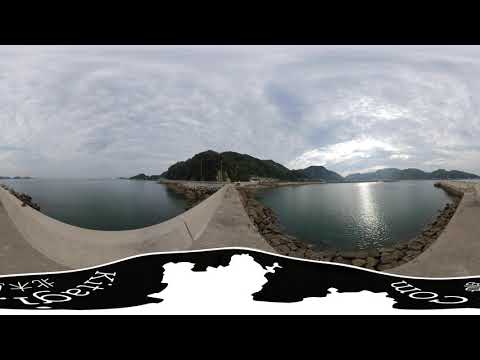The image presents a panoramic, slightly distorted view of a long concrete pier extending from the shoreline into a calm, dark blue body of water. The pier, flanked by large rocks forming sea defenses, leads out towards a mountainous island with a rugged, craggy outline. In the distance, more hills and mountains can be seen stretching across the horizon. The pathway of the pier runs down the center of the image, bordered by a low wall on the left and curving around into the water in a U shape to the right. The sky above is a mix of overcast clouds and intermittent sunlight, particularly bright on the right side, casting a reflective light on the tranquil water below. In the foreground, text appears upside down, reading "KITAGI" on the left and "COM" on the right, possibly part of a map or sign. The vantage point suggests the image might have been taken from the top of a person's head, contributing to its unique perspective.